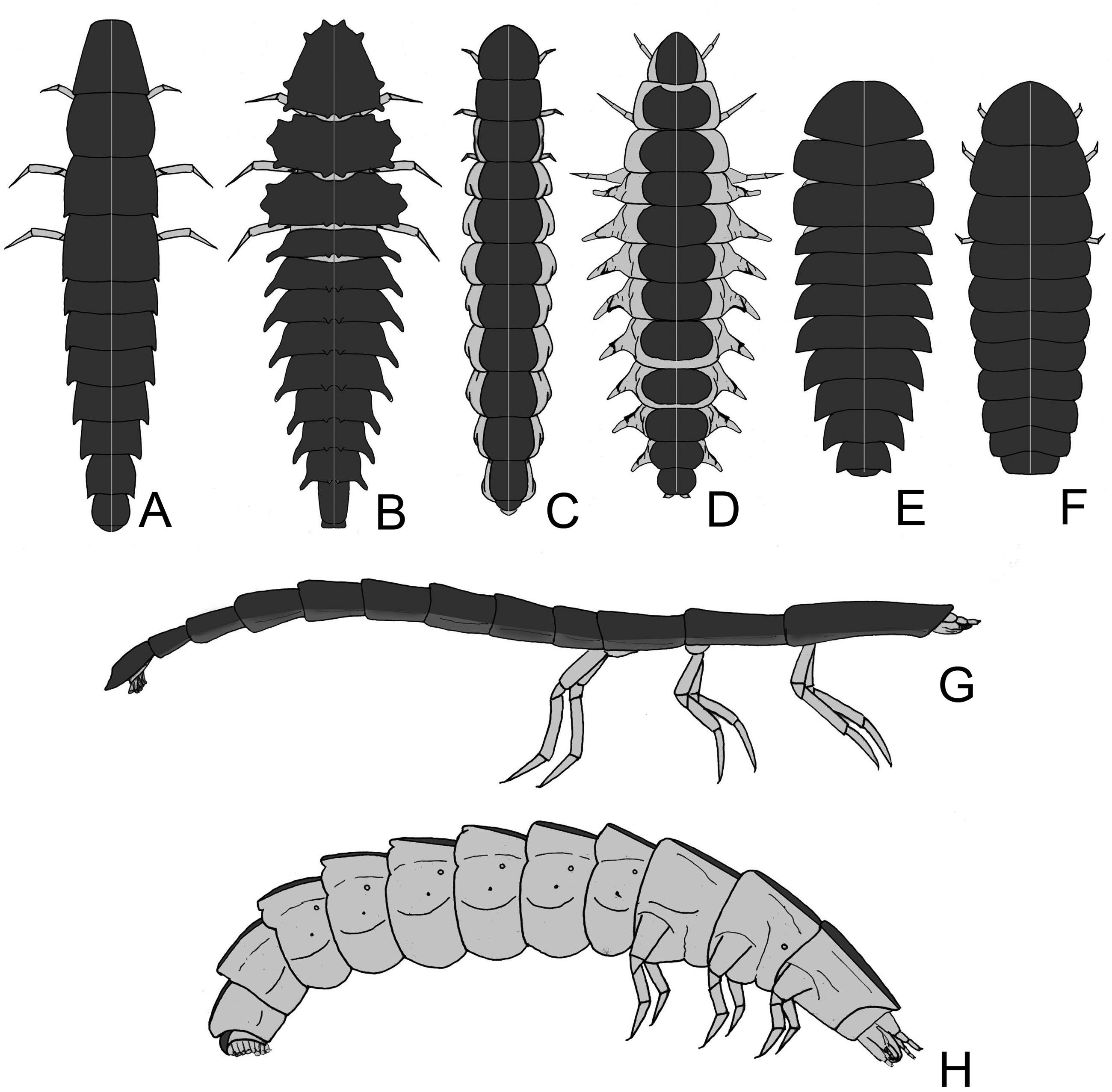This image is a detailed, black-and-white chart illustrating various multi-segmented bugs or arthropods, laid out in a structured format. The top row consists of six images labeled A, B, C, D, E, and F, depicting the dorsal (top) views of different insects or similar creatures. Below these, there are two additional images: an elongated bug labeled G, shown from the left-hand side, and another slightly raised in position, labeled H, also viewed from the left-hand side. All illustrations are in grayscale, allowing for clear visibility of each insect's segmented body and varying number of legs, providing a comprehensive study of these arthropods' external structures.